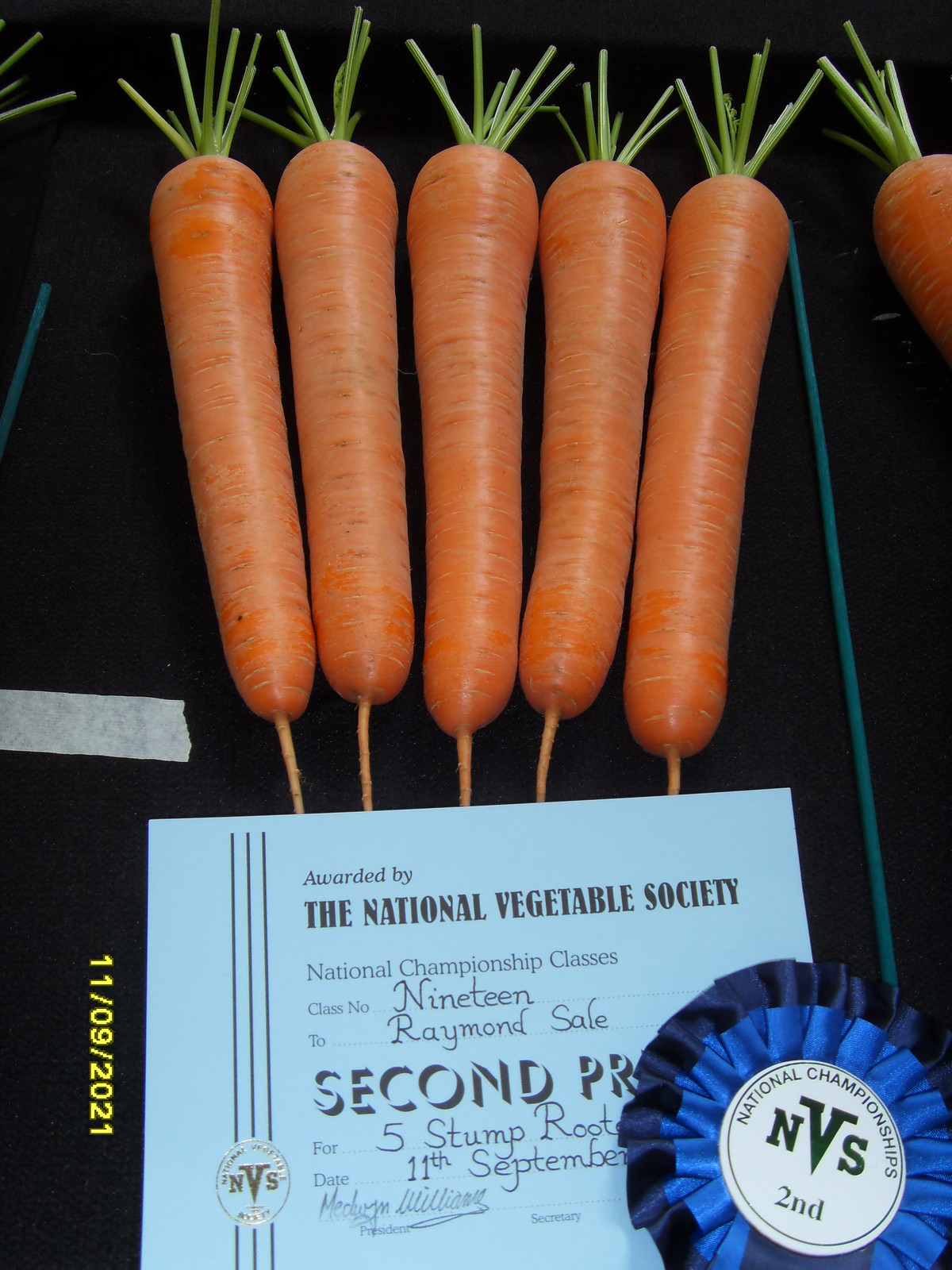The image is a detailed photograph showcasing five nearly identical carrots arranged in a vertical position on a black tablecloth. Each carrot has been trimmed, leaving about an inch of the green top intact, and still retains some roots at the bottom. Beneath the carrots lies a blue certificate that reads "Awarded by the National Vegetable Society, National Championship Classes, Class No. 19 to Raymond Sale, second prize," dated 11th September 2021. In the lower right-hand corner, a blue ribbon with green lettering displays "National Championships, NVS, second place." The certificate also has a signature believed to be Meadwin Williams, adding an official stamp to Raymond Sale's accomplishment in class number 19 for "five stump-rooted carrots."